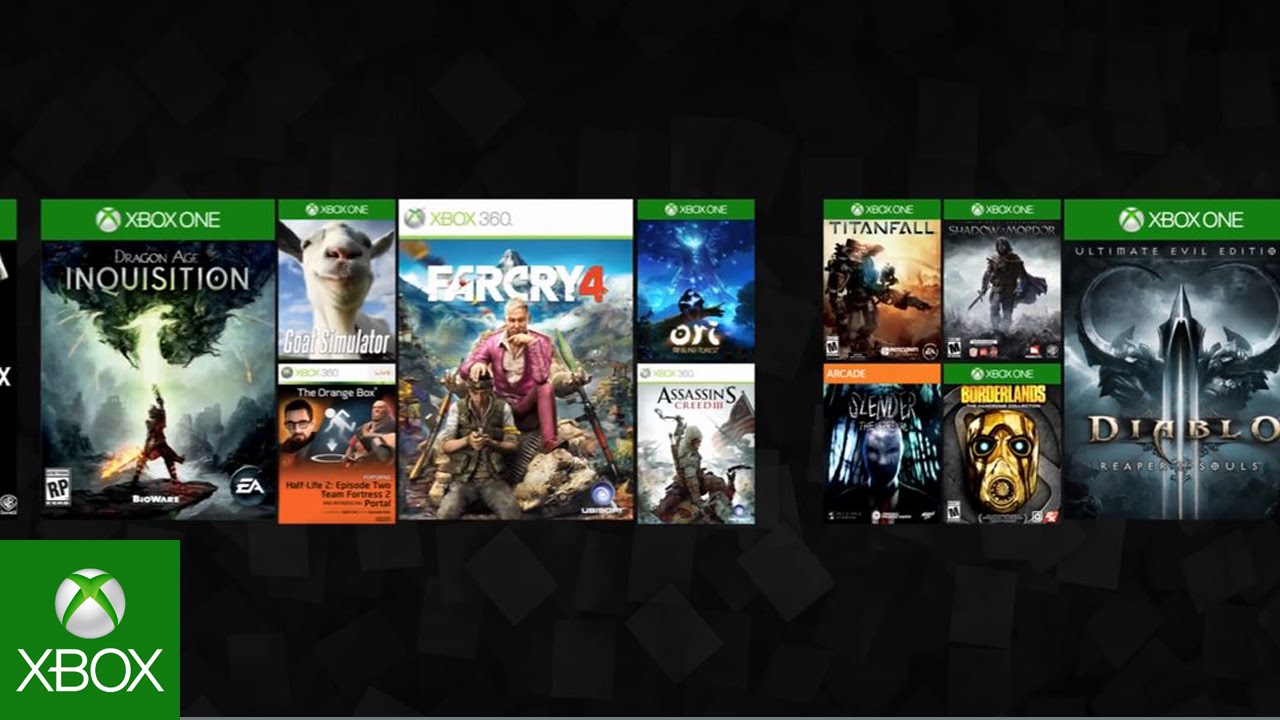The image displays a rectangular screen with a black background, showcasing a variety of Xbox-related banners. In the lower left corner of the screen, there is a green square featuring the Xbox logo and the word "Xbox" in white lettering. 

Starting from the left, the first banner spans the full width and displays the title "Inquisition." The next section is split into two images stacked vertically. The top image is labeled "Goat Simulator," while the bottom one shows a person and an outline of a falling person beside another figure, but the text is unclear, possibly reading "The Orange Room." 

Following this, there is a full-length banner titled "Far Cry 4." Continuing, another vertically split section features "Ork" on the top image and "Assassins" on the bottom. 

Further to the right, after a section of black space, there are two more images stacked vertically: the top one labeled "Titanfall" and the bottom one labeled "Slender." Adjacent to this, there are two images side by side, with the bottom one clearly showing "Borderlines." 

The sequence concludes with a full-width banner titled "Diablo."